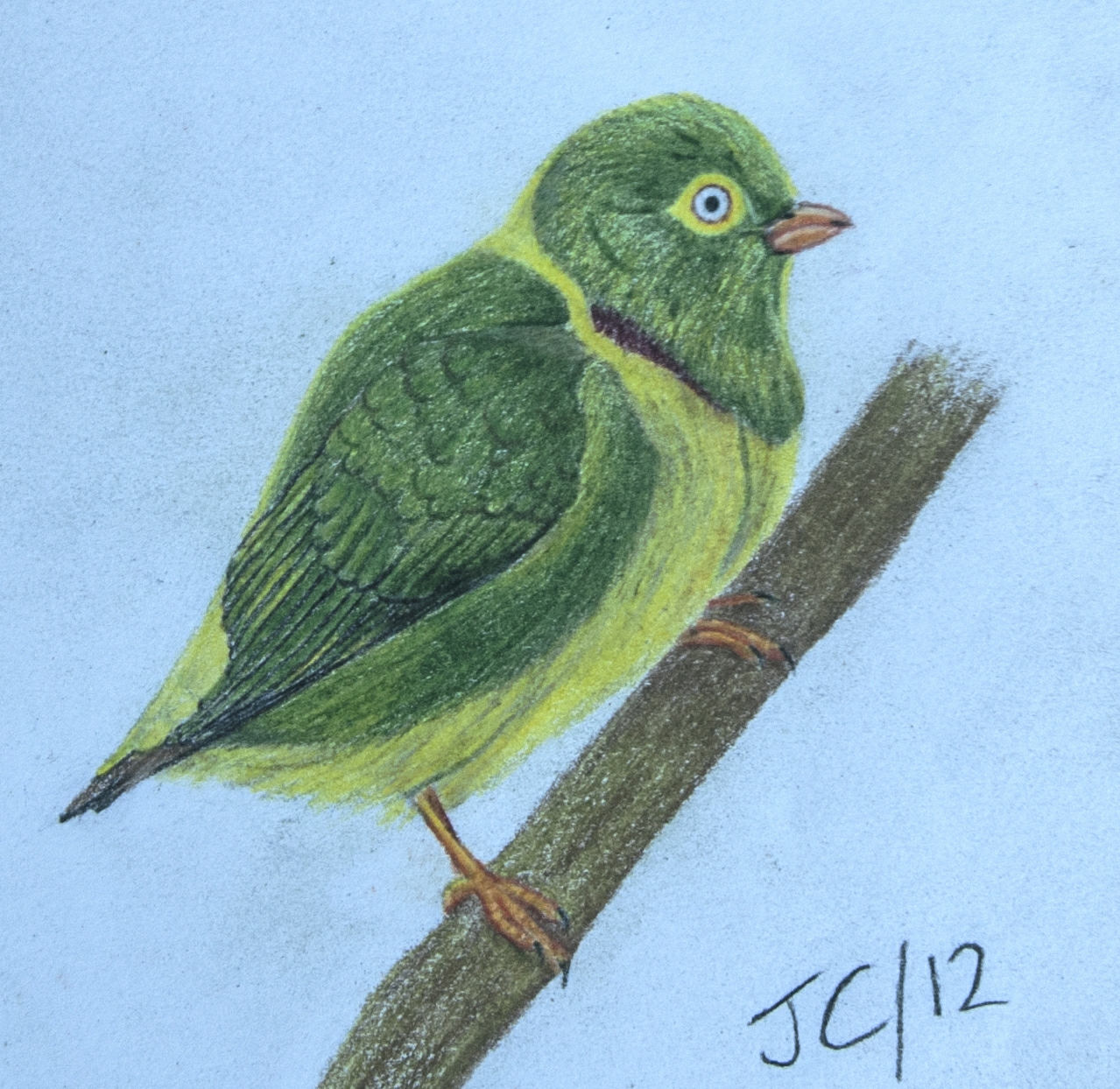A meticulously drawn bird is perched gracefully on a branch in this illustration. The bird, displaying vivid green plumage, is clutching the branch firmly with its sharp claws. Its head is also green, accentuated by a striking yellow beak. Yellow feathers encircle its eyes, creating a distinctive appearance. Just below its green feathers, there is a touch of black, adding contrast to its vibrant coloration. The bird's belly is a bright yellow, and this yellow hue extends around its neck and along its back. Its back feathers also exhibit this yellow tone. The bird's wings are primarily green with hints of black and small white specks scattered through both its wings and head. The background is a soft, powder blue, providing a serene setting for the vivid colors of the bird. At the bottom right corner of the drawing, the text "JC/12" is inscribed.